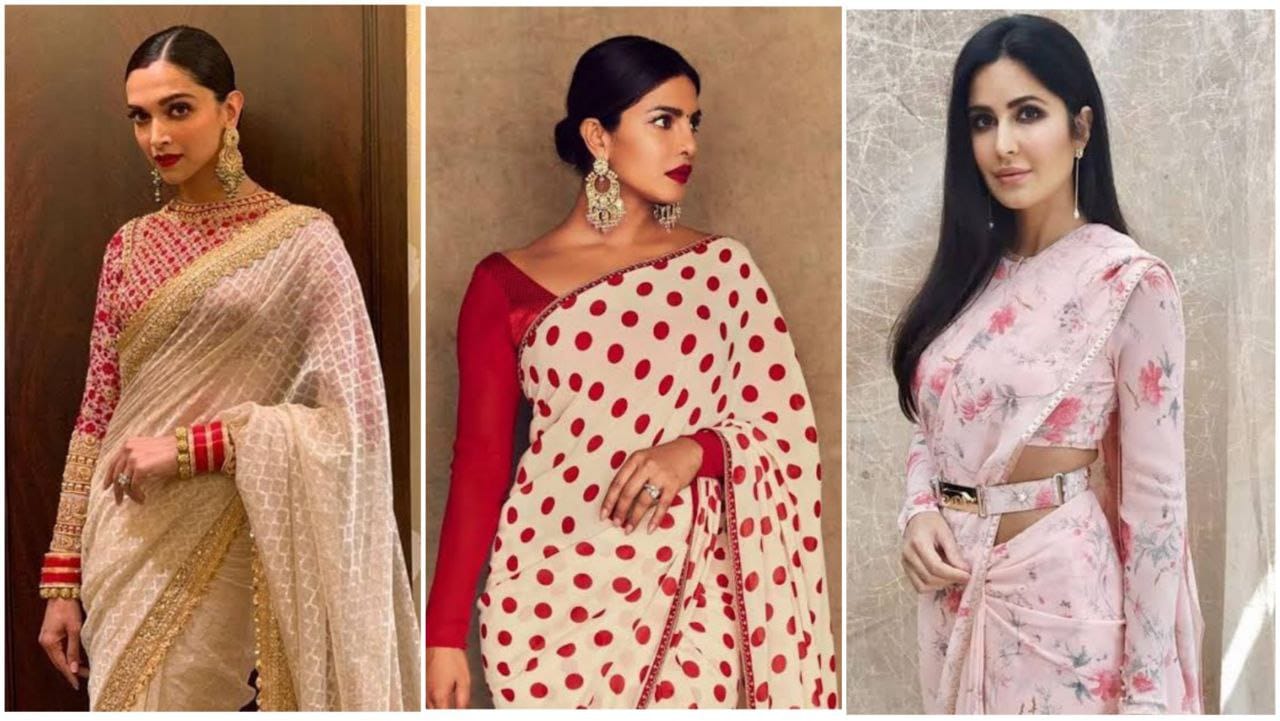This composite image features three Indian women in traditional attire. Each woman is photographed individually, and the photos are aligned side by side. 

On the left, the woman has her hair slicked back and sports large earrings. She wears a luxurious sari with a geometric design in pink, gold, and white. She also has bracelets on her wrist. 

The central woman has her black hair styled in a bun, complemented by large gold earrings and bright red lipstick. She wears a sari with a pink and white polka-dot pattern, accessorized with a single red sleeve on her left arm.

Finally, the woman on the right has long, straight black hair cascading down. She wears a white sari adorned with pink floral designs and a golden belt buckle. She completes her look with pendant earrings.

All three women face slightly off to the side, showcasing their sophisticated and culturally rich ensembles.